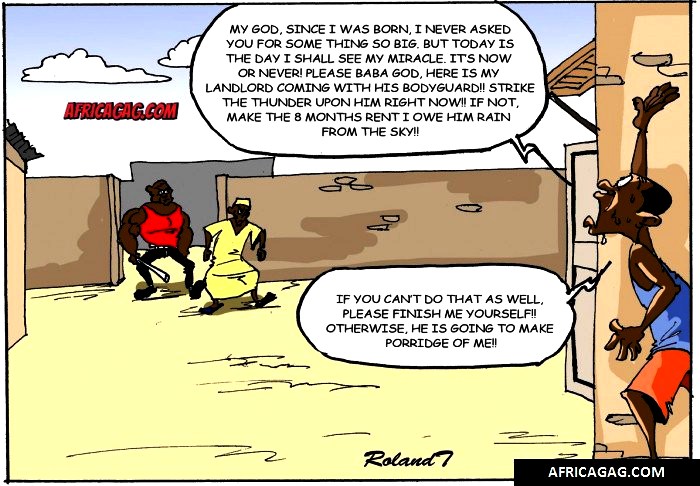In a single, vividly detailed comic frame from AfricaGag.com, a blue sky with white clouds serves as the backdrop. On the bottom right, a black rectangle with white lettering prominently displays "AfricaGag.com." Nearby, in cursive writing, the word "Roland" appears, though one character remains indistinct.

To the right side of the frame, a dark-skinned man, sweating and visibly distressed, stands with his right hand raised and his left hand splayed out in front. He wears a dark blue tank top paired with orange knee-length shorts. His speech bubble reads, "My God, since I was born, I never asked you for something so big, but today is the day I shall see my miracle. It's now or never, please Baba God. Here is my landlord coming with his bodyguards. Strike the thunder upon him right now. If not, make the eight months rent I owe him rain from the sky. If you can't do that as well, please finish me yourself. Otherwise, he is going to make porridge of me."

Emerging through an entrance in a brown wall, with a yellow ground beneath them, are two intimidating figures. One is a muscular black man wielding a weapon that might be a sword, machete, or baseball bat in his right hand. He wears a gray tank top. Beside him is another dark-skinned man dressed in a yellow robe and matching shorts with a small white hat. The landlord and his bodyguard stride menacingly towards the desperate man, enhancing the comic's tension and highlighting its humorous plea for divine intervention.